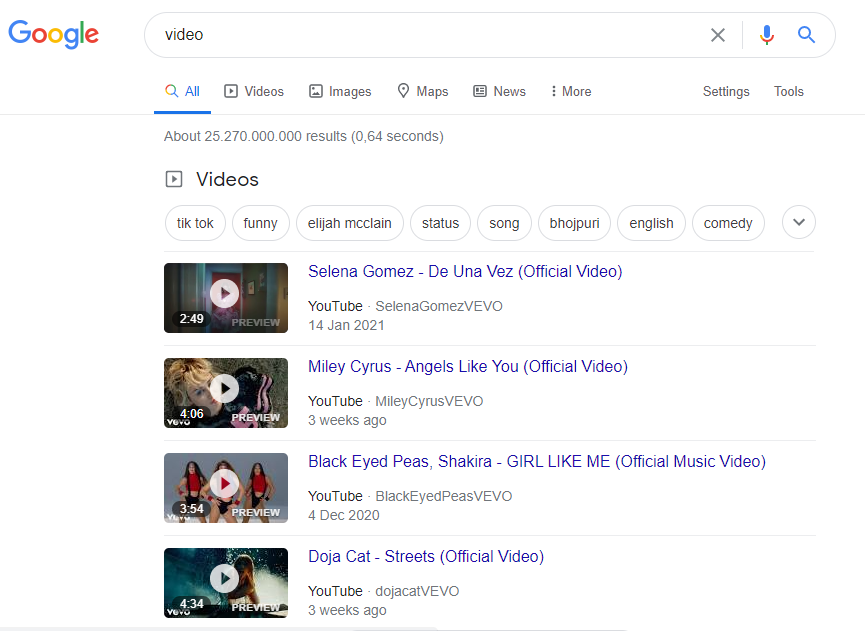The image displays a Google search results page. In the top left corner, the iconic "Google" logo is clearly visible. To the right of the logo is a search bar with the keyword "video" entered. Adjacent to the search bar, on the right, are an "X" icon for clearing the search, a microphone icon for voice search, and a search button.

Directly beneath the search bar, the category "All" is highlighted in blue, indicating that it is the currently selected filter. The other categories—Videos, Images, Maps, News, More, Settings, and Tools—are grayed out, shown sequentially from left to right.

Below these categories, the page displays the search result count, which reads approximately "25,270,000,000 results." The results section below lists video-related searches, including popular queries such as "TikTok funny," "Elijah McClain," "status," "song BHO JP URI," "English comedy," and a category represented by a circle with a downward arrow.

The main content includes four video search results, all sourced from YouTube:
1. **Selena Gomez - "De Una Vez"** (2 minutes 49 seconds)
2. **Miley Cyrus - "Angels Like You"** (4 minutes 5 seconds)
3. **Black Eyed Peas & Shakira - "Girl Like Me"** (3 minutes 54 seconds)
4. **Doja Cat - "Streets"** (4 minutes 34 seconds)

Each result features the video's title, artist, and duration, providing a succinct overview of the content available under the searched term "video."